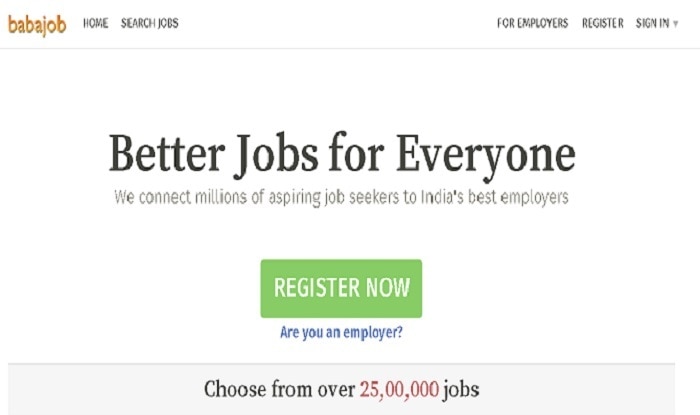This screenshot captures a section of the "BABA Job" website. In the upper left corner, the site’s name, "BABA Job," is prominently displayed. At the top of the page, there are navigation buttons organized in two groups: on the left, "Home" and "Search Jobs," and on the right, "For Employers," "Register," and "Sign In." Central to the page is a bold headline stating, "Better Jobs for Everyone," followed by a subtext that reads, "We connect millions of aspiring job seekers to India's best employers." Below this, there's a prominent green button labeled "Register Now" in white text. Slightly beneath this button, in blue text, a clickable option says, "Are You an Employer?" At the very bottom, a section declares, "Choose from Over 25 Million Jobs," where "25 Million Jobs" is highlighted in red text, contrasting with the black text used for the rest of the sentence. This section is set against a darker gray background, providing a clear visual distinction from the rest of the page.